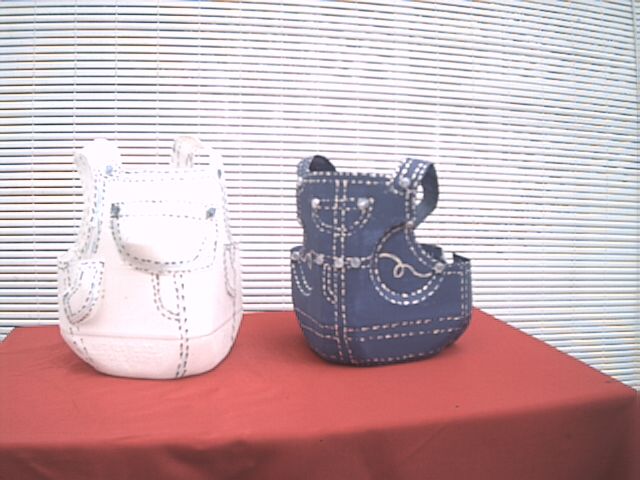The image depicts two sculptural pieces that resemble overalls, positioned on a small table draped with a red cloth. These objects could be mistaken for purses or backpacks due to their intricate design and functionality features. The sculpture on the left is white with dark blue stitching and appears tall and sturdy. It features stud-like accents and detailed fake pockets. The sculpture on the right mimics denim overalls with a blue coloration, white stitching, and a similar design of studs and pockets, giving an illusion of utility. Notably, this sculpture also has an open, bowl-like back. Both sculptures stand out brightly against the red tablecloth, illuminated by the light filtering through the long, mini window blinds in the background, which adds to the vividness of the scene.